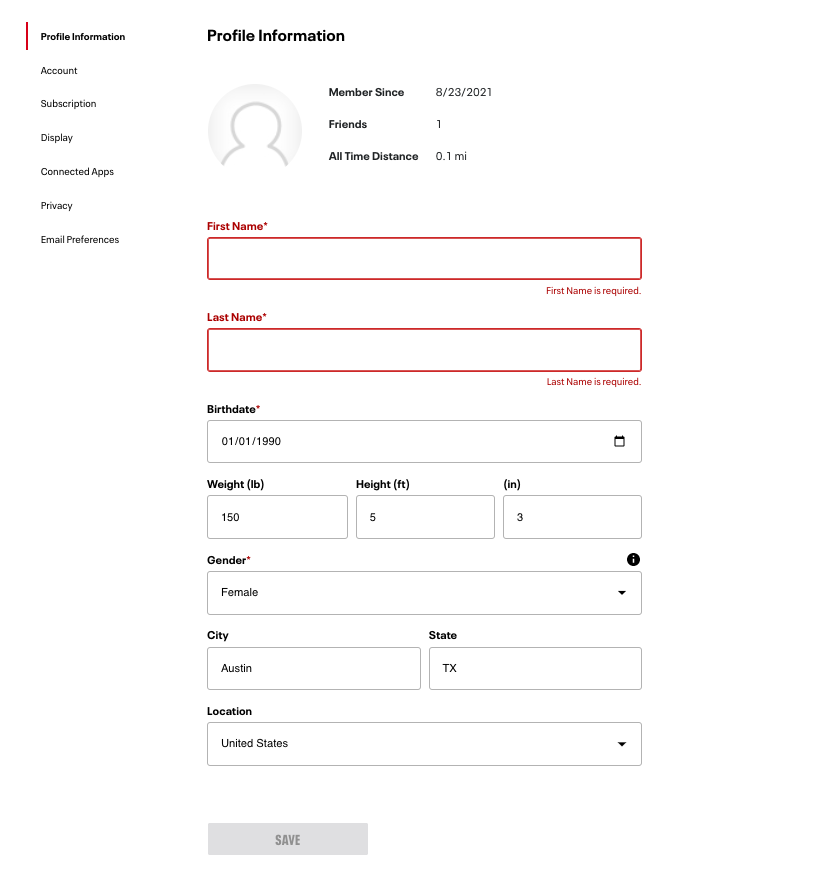Here is a cleaned-up and detailed caption for the given image:

---

The webpage is designed to collect profile information and features a predominantly white background with small black text for clarity. At the top-left corner of the white box, navigation links are labeled: "Profile Information," "Account," "Subscription," "Display," "Connected Apps," "Privacy," and "Email Preferences." Centrally positioned at the top in bold, "Profile Information" denotes the section's focus. 

Below, there’s a placeholder space for a profile picture, alongside membership details reading, "Member since 08-23-2021," "Friends: 1," and "All-time distance: 0.1." 

Further down in the middle of the page, a red box with red text draws attention to required fields. The sections include:
- "First Name" with an adjacent note indicating it is required.
- "Last Name" likewise noted as required.
- "Birth Date: 01-01-1990."
- "Weight: 150 pounds."
- "Height: 5 feet 3 inches."
- "Gender: Female."
- "City: Austin."
- "State: Texas."
- "Location: United States."

At the very bottom of the form, a grayed-out "Save" button awaits completion of the fields before activation.

Overall, the webpage's bright white backdrop contrasts effectively with the small black text, ensuring readability of the detailed profile information fields. Completion of the form allows the user to save their details via the save button.